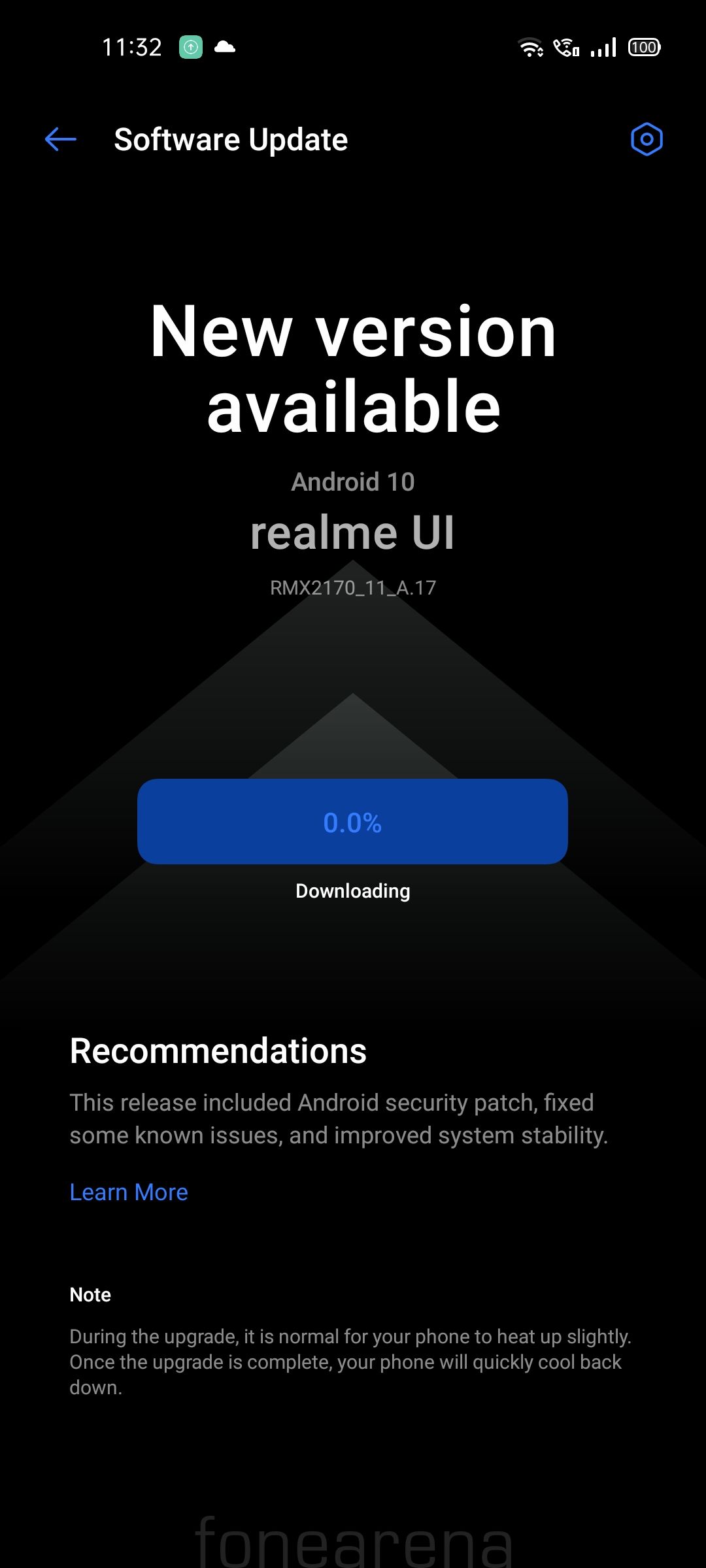The image depicts a smartphone screen featuring a software update notification against a black background. The top right corner displays the current time, 11:32, highlighted in white with a green box adjacent to it. To the right, three cell phone signal bars are visible, increasing in height as they curve upwards, followed by a battery symbol.

Below this, a white text indicates "Software Update," accompanied by a blue left-pointing arrow to the left and a small blue circle. Centrally positioned is the text "New Version Available: Android 10" in white, immediately followed by "Realme UI" in uppercase letters.

A large light gray triangle, wide at the base, is situated beneath the text. Directly below the triangle is a long blue rectangle reading "0.0%," with the word "Downloading" in white text underneath. Further down, in white text, it states "Recommendations: This release includes Android security patch, fixes known issues, and improves system stability." The phrase "Learn More" is written in blue text at the very bottom.